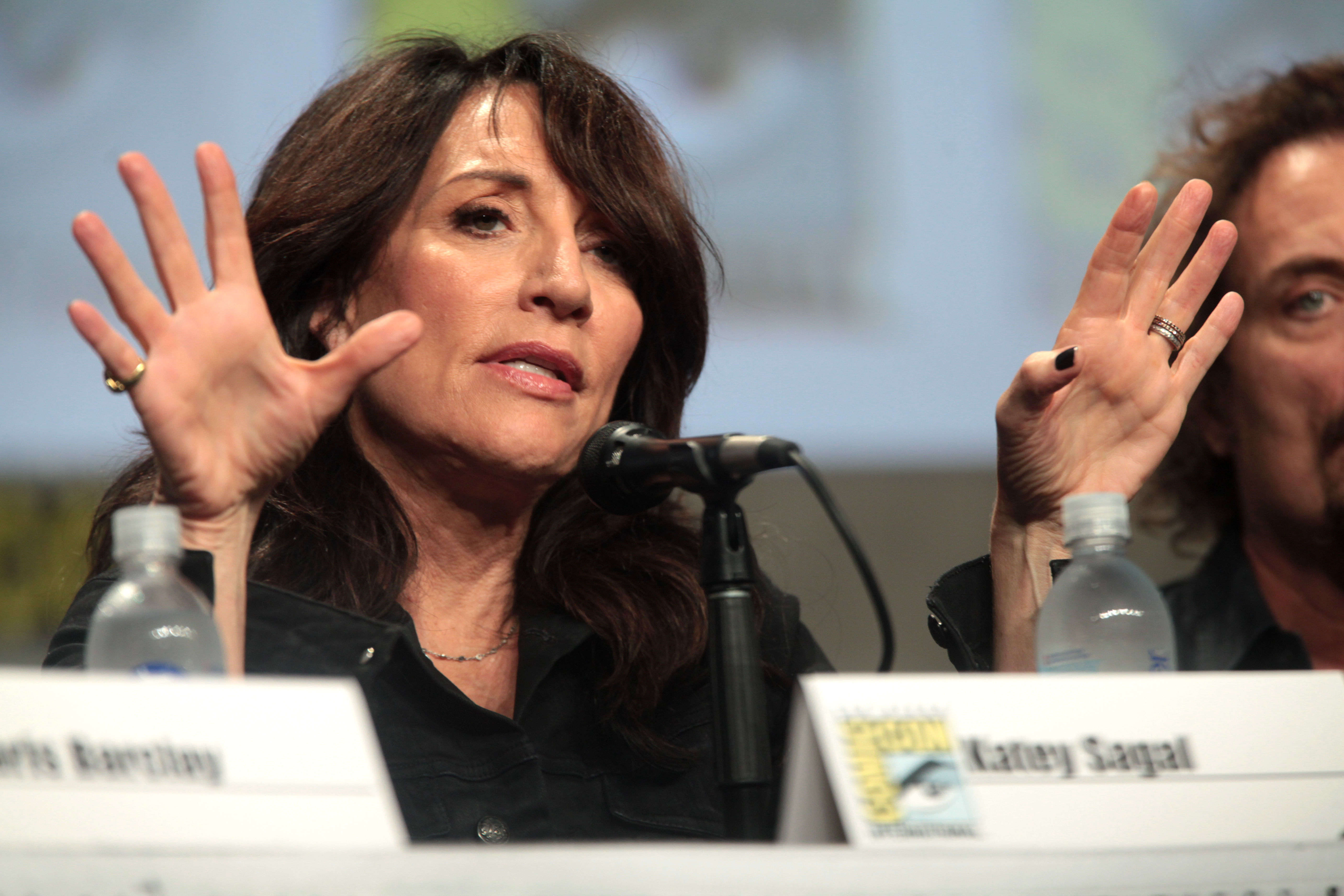In the image, actress Katie Seagal is seated at a podium behind a microphone, gesturing with both hands raised and her palms facing forward. She has long brown hair that falls just below her neck, partially covering one eye, and wears black nail polish with a distinct detail of a painted thumbnail on her left hand. Katie is adorned in a black blouse resembling a jean jacket with button details, complemented by a slim necklace and a small ring on her right pinky finger. A name tag with “Katie Seagal” prominently sits in front of her in a V-shape, while another blurred name tag is to its left. The background is blurred, adding focus to Katie and partially to a man next to her with curly, slightly wild hair and a faint mustache. The podium is shared with him, along with visible water bottles, suggesting they are part of the same panel discussion or event.